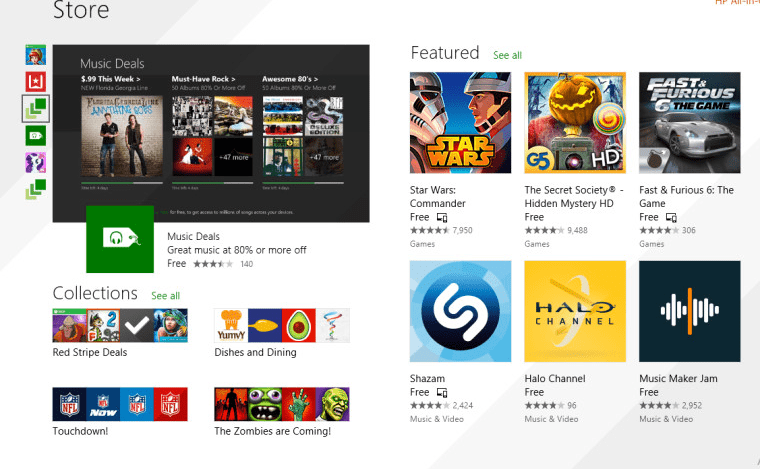This image captures a screenshot of what appears to be the Microsoft App Store interface. The background is predominantly white with subtle gray shading in the top left and lower right corners. 

In the top left corner, the word "Store" is prominently displayed. Directly below it, a small black box reads "Music Deals," showcasing various album covers beneath it. Below the albums, a green box announces, "Music Deals: Great music at 80% or more off."

Continuing downward, there is a "Collections" section that includes several categories: "Red Stripe Deals," "Dishes and Dining," "Touchdown," and "The Zombies are Coming."

Occupying a significant portion of the page to the right is the "Featured" section, which highlights six applications. These include:
1. Star Wars Commander
2. Secret Society - Hidden Mystery
3. Fast & Furious 6: The Game
4. Shazam
5. Halo Channel
6. Music Maker Jam

This descriptive display provides a concise overview of the various deals, collections, and featured applications available in the Microsoft App Store.